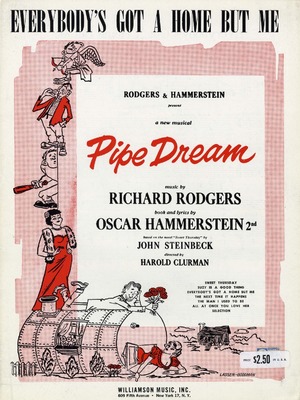This poster is an evocative vintage illustration with rich and intricate details. Dominated by a large central white rectangle bordered in white and enveloped within a reddish hue, it prominently features the title "Everybody's Got a Home But Me" written in bold black at the top. Beneath the title, it proudly announces "Rodgers and Hammerstein present Pipe Dream," with music by Richard Rodgers and lyrics by Oscar Hammerstein II. Details continue with the mention of "John Steinbeck" and direction by "Harold Klurman."

On the left side, an artistic assembly of figures populates a pink plaid background. These include a Cupid-like angel rendered in black ink with a bow and arrow, a man attired in a striking red coat and white pants, and a caveman brandishing a wooden club. Below them, a woman in a flowing red dress with a fur stole around her neck stands gracefully. She has black hair and is perched atop a large, round pipe or submarine. A man in a white coat lies on this pipe, holding a bouquet of red roses towards another woman in a red dress, who is reclined inside the pipe. The price "$2.50" appears discreetly in black at the bottom right.

This beautifully detailed illustration captures a whimsical and nostalgic essence, reflecting the charm and intricacies of mid-20th century poster art.